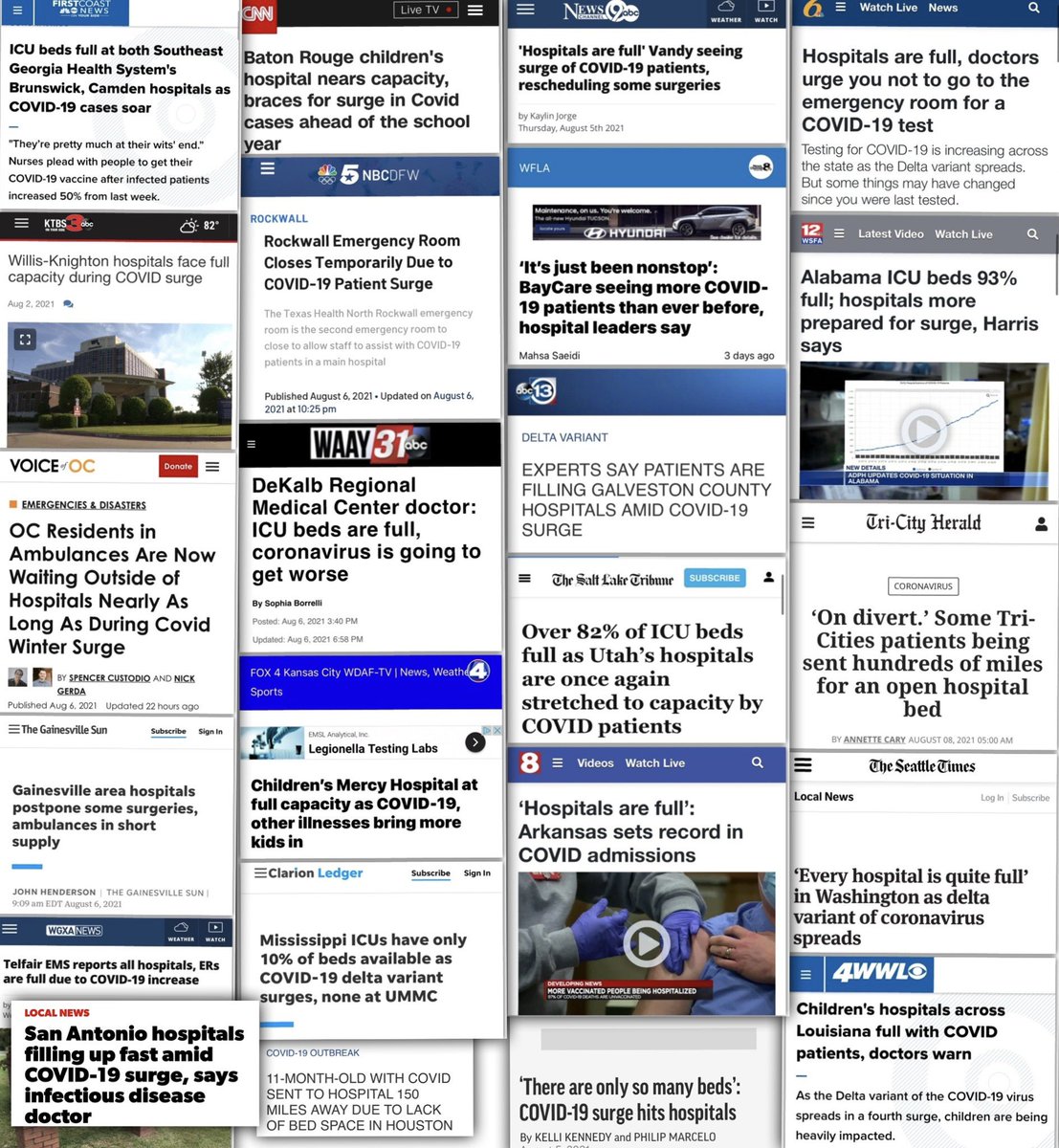In this image, there is a collage of news headlines and articles showcasing the intense strain on hospitals across various regions due to the COVID-19 pandemic. The headlines focus on multiple hospitals, including Southeast Georgia Health Systems' Brunswick and Camden locations, which report that their ICU beds are at full capacity as COVID-19 cases rise significantly. 

Nurses are depicted pleading with the public to get vaccinated as they face overwhelming numbers, with infected patient numbers having increased by 50% in just a week. Baton Rouge Children's Hospital is highlighted for nearing full capacity, preparing for a further surge in cases. Similarly, Vanderbilt University Medical Center is shown grappling with a growing influx of COVID-19 patients, leading to the rescheduling of some surgeries. 

The articles emphasize that hospitals are urging the public not to visit emergency rooms solely for COVID-19 tests, as testing demand escalates due to the Delta variant's spread. Orange County residents are described waiting in ambulances outside hospitals for extended periods, reminiscent of the previous winter surge.

Additionally, statements from Brickhub Regional Medical Center indicate that ICU beds are entirely occupied, with dire predictions that the situation will worsen. The collage also spotlights Galveston County hospitals experiencing similar strain and Utah hospitals where over 80% of ICU beds are filled, pushing facilities to their limits once again.

This compilation powerfully illustrates the urgent and ongoing healthcare crisis, with medical professionals and experts repeatedly calling for public vaccination and caution as the pandemic persists.